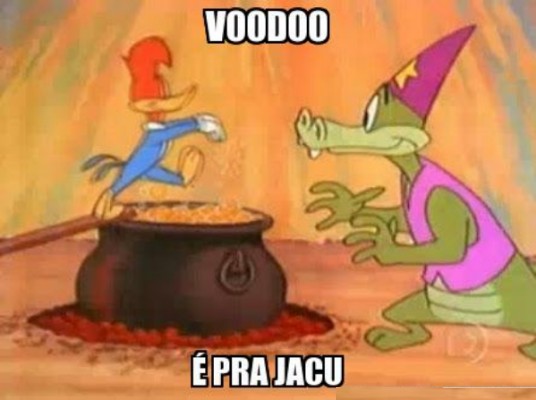In this vivid cartoon meme, Woody Woodpecker is portrayed on the left, seemingly under a spell as he walks, eyes closed and arms extended, off a plank into a large black cauldron of boiling orange liquid. Steam rises from the cauldron, indicating its heat. Woody has his classic red head, yellow beak, blue body, white gloves, and yellow feet, with one foot already above the bubbling pot and the other still on the plank.

On the right side of the image, a green anthropomorphic alligator stands on its hind legs, observing Woody with a greedy expression. This alligator character is dressed in a pink vest and a purple beanie adorned with a gold star. Two teeth protrude from the corners of its mouth just below the nose.

The detailed background includes a brown floor under the cauldron and text that adds context: the word "voodoo" is prominently displayed at the top, while the bottom features text in Portuguese, “é pra jacu,” written in white letters with a black outline. The scene suggests a spell or magical ritual, with the alligator character eagerly anticipating Woody's plunge into the mystical brew.